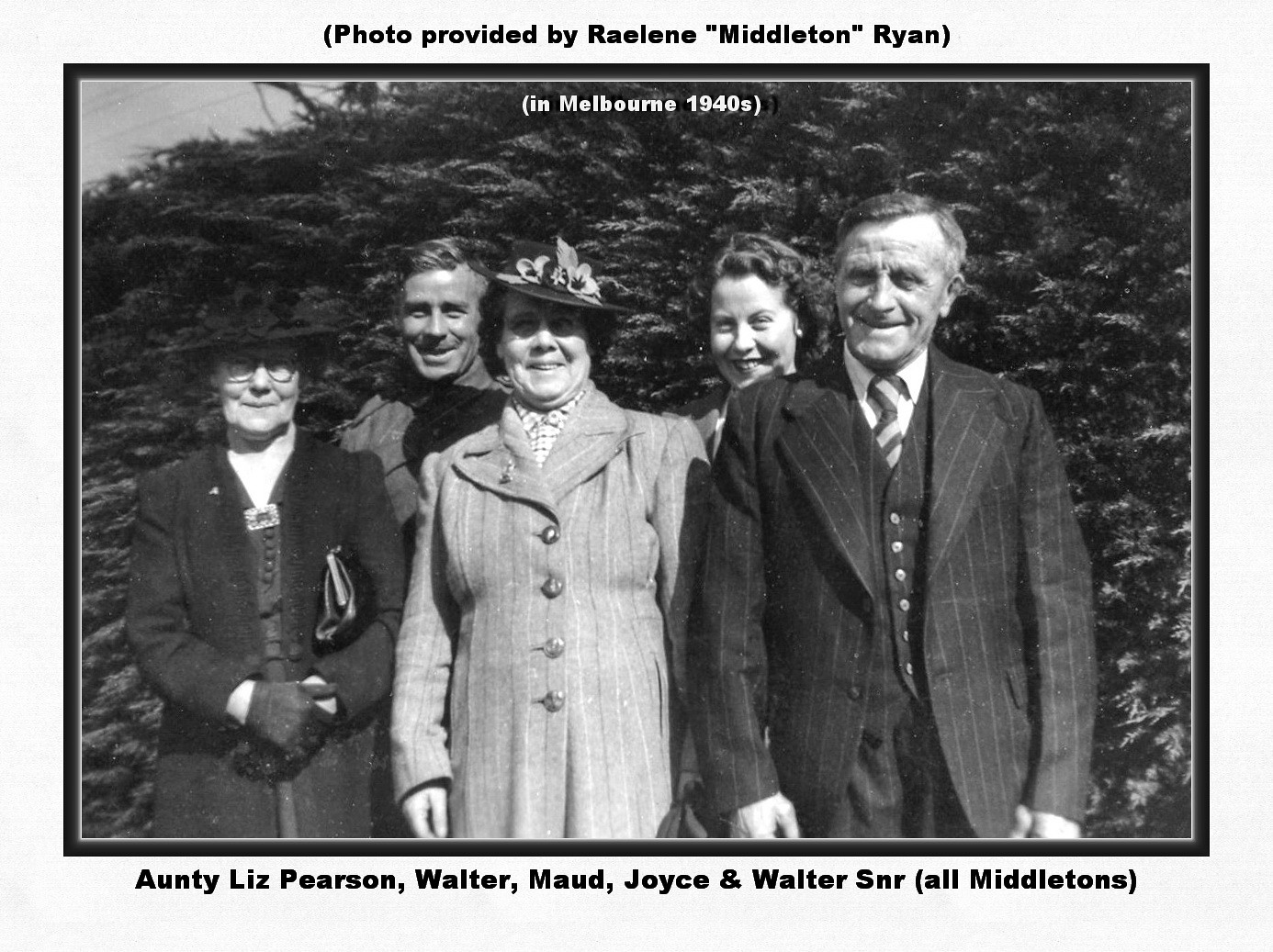The photograph, provided by Raylene "Middleton" Ryan, captures a historical 1940s family gathering in black and white. It depicts five elderly individuals, all smiling and posing against a lush backdrop of bushes and trees on a gray, possibly chilly Melbourne day. At the top of the image, a watermark in white text reads, "in Melbourne, 1940s." The group consists of three women and two men, dressed in period-appropriate attire; the women are wearing button-up coats and hats adorned with flowers, one even sporting gloves. Among the men, one appears to be in a soldier’s uniform. Above the image, black text credits Raylene Middleton Ryan. Below, another caption identifies the individuals as Auntie Liz Pearson, Walter, Maud, Joyce, and Walter Sr., all members of the Middleton family. The top left corner of the image faintly shows three black lines, possibly telephone or electrical poles, adding a subtle hint of infrastructure to the pastoral scene.